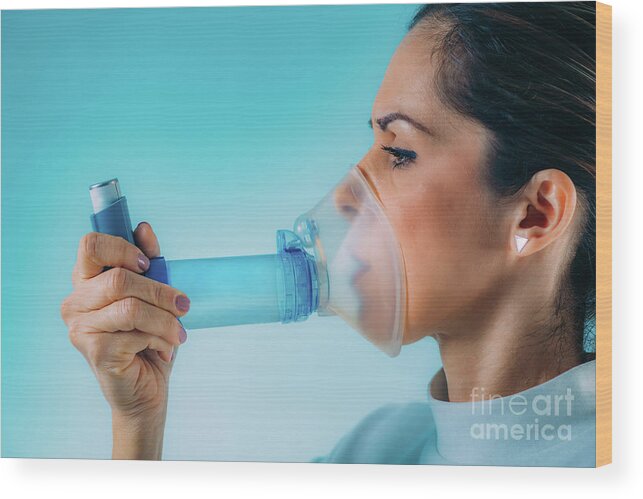The image features a detailed close-up of an older woman, likely in her fifties, viewed in profile with her left side turned towards the viewer. She has her brown hair tied back and is wearing white triangular stud earrings. Her attire consists of a light blue, possibly turtleneck, sweater. The woman is holding a blue medical inhaler in her right hand, which is connected to a respirator mask covering her nose and mouth via a light blue tube. The inhaler is depicted in the left third of the image, while the woman's face occupies the right third. The background is a gradient light blue, adding to the clinical feel of the scene, which resembles material from a hospital instruction manual or medical guidebook. In the lower right-hand corner of the image, the text "Fine Art America" is visible, likely indicating the stock photo source.